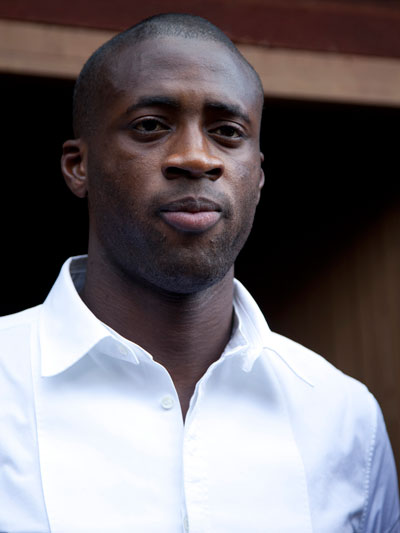In the image, a black male with brown eyes and very short hair has a subtle presence with a touch of black stubble on his face. His age appears to be in the mid-30s, discernible from the light lines on his forehead. His expression is neutral with closed lips, and he seems to be looking slightly past the photographer rather than directly at the camera. The man is dressed in a bright white button-up collared shirt that looks very clean and well-pressed, featuring a large collar and slightly open neck revealing part of his upper chest. The background behind him is blurred and predominantly brown with light tan and black hues, adding a soft contrast that keeps the focus on him. The photo is centered on the man, capturing him from chest level upwards, and the setting leaves it ambiguous whether it’s taken indoors or outdoors.